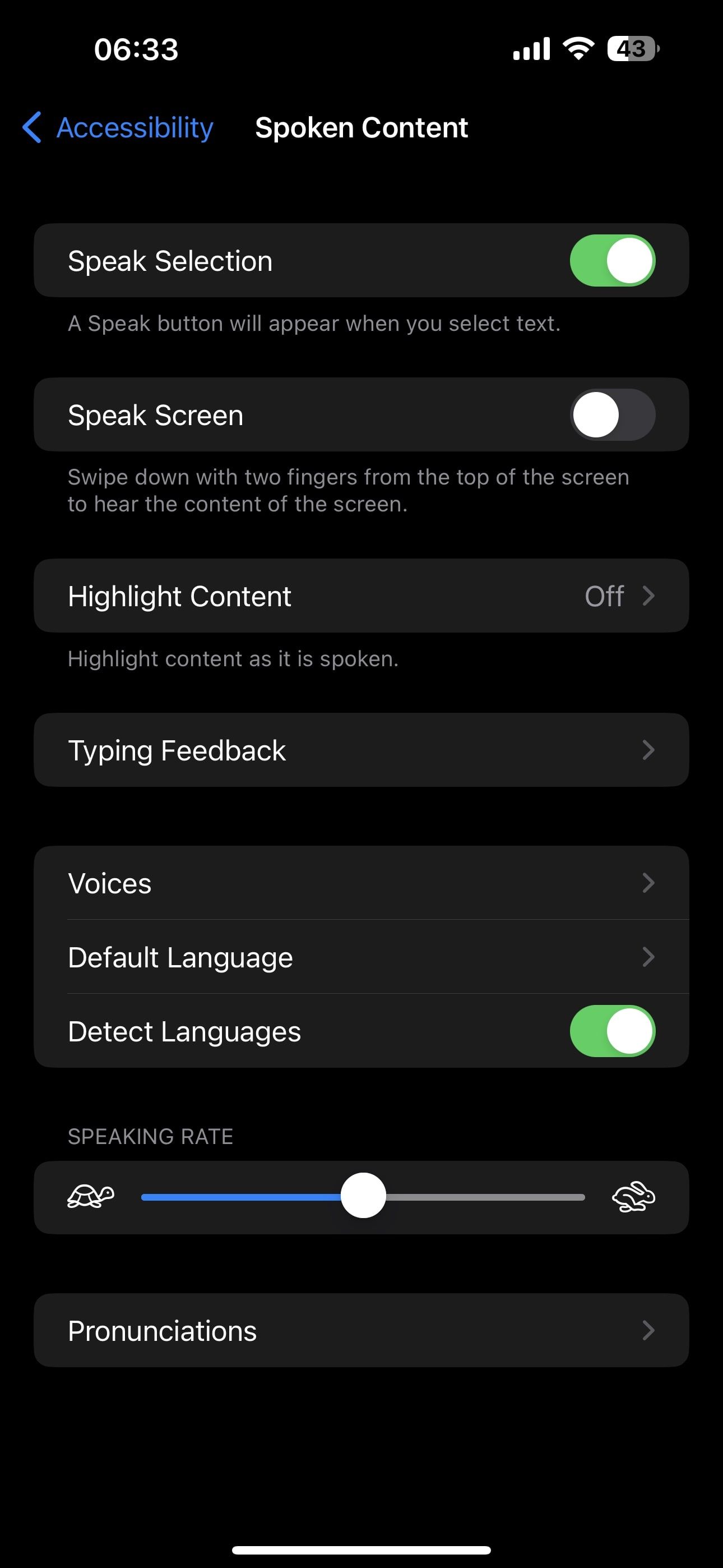This image is a screenshot of a cell phone screen with a black background. 

In the upper left corner, the time is displayed as "06:33", with the numbers separated by a colon. Moving to the right, there are four vertical bars indicating cellular signal strength, and the battery icon shows 43% charge, with half of the icon filled in white.

Below this section, there is a small blue arrow pointing left, next to the word "Accessibility" in blue text. To the right of this, in white text, it says "Spoken Content".

The next line reads "Speak Selection", with a white circle positioned to the right within a green area, indicating that it's turned on. Below it, "Speak Screen" is labeled, with a white circle to the left outside of the green area, showing that this feature is not activated.

The following section is "Highlight Content", which is turned off. "Typing Feedback" is listed next, followed by an arrow pointing right, suggesting more options.

Next, "Voices" is displayed with "Default" next to "Language", and "Detect Languages" has a white circle to the right of a green area, indicating it’s turned on. 

The "Speaking Rate" section features a turtle icon on the left, a rabbit icon on the right, and a white circle in the center of the line, signifying a medium speaking rate.

Finally, at the bottom, the word "Pronunciations" appears with a small arrow pointing right, implying additional settings or options.